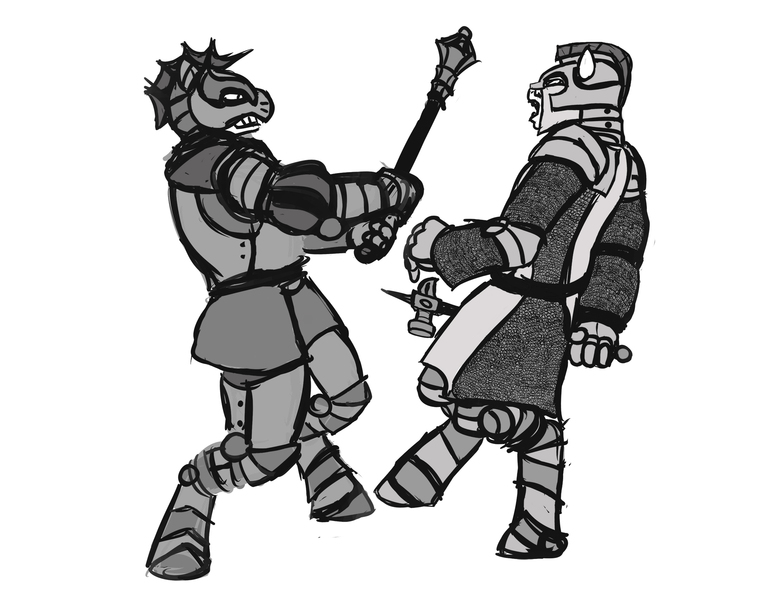The black-and-white digital illustration depicts a dynamic duel between two anthropomorphic characters, accentuated by intricate details and grayscale shading. On the left, a character with a wolf-like head, clad in medieval-style plate armor with visible rivets, wields a spiked staff, swinging it menacingly. The character sports a distinctive mohawk resembling a dragon wing. On the right, a similarly armored figure, identified by a metal helmet adorned with a mohawk spike, brandishes a mace-like weapon with a hammer-like edge. This character’s open mouth reveals sharp teeth, and their armor primarily consists of chainmail covering the torso, complemented by metal protection for the elbows, knees, and feet. Both combatants are engaged in an intense fight, set against a pure white background devoid of any text or signatures, enhancing the stark contrast and clarity of the scene.